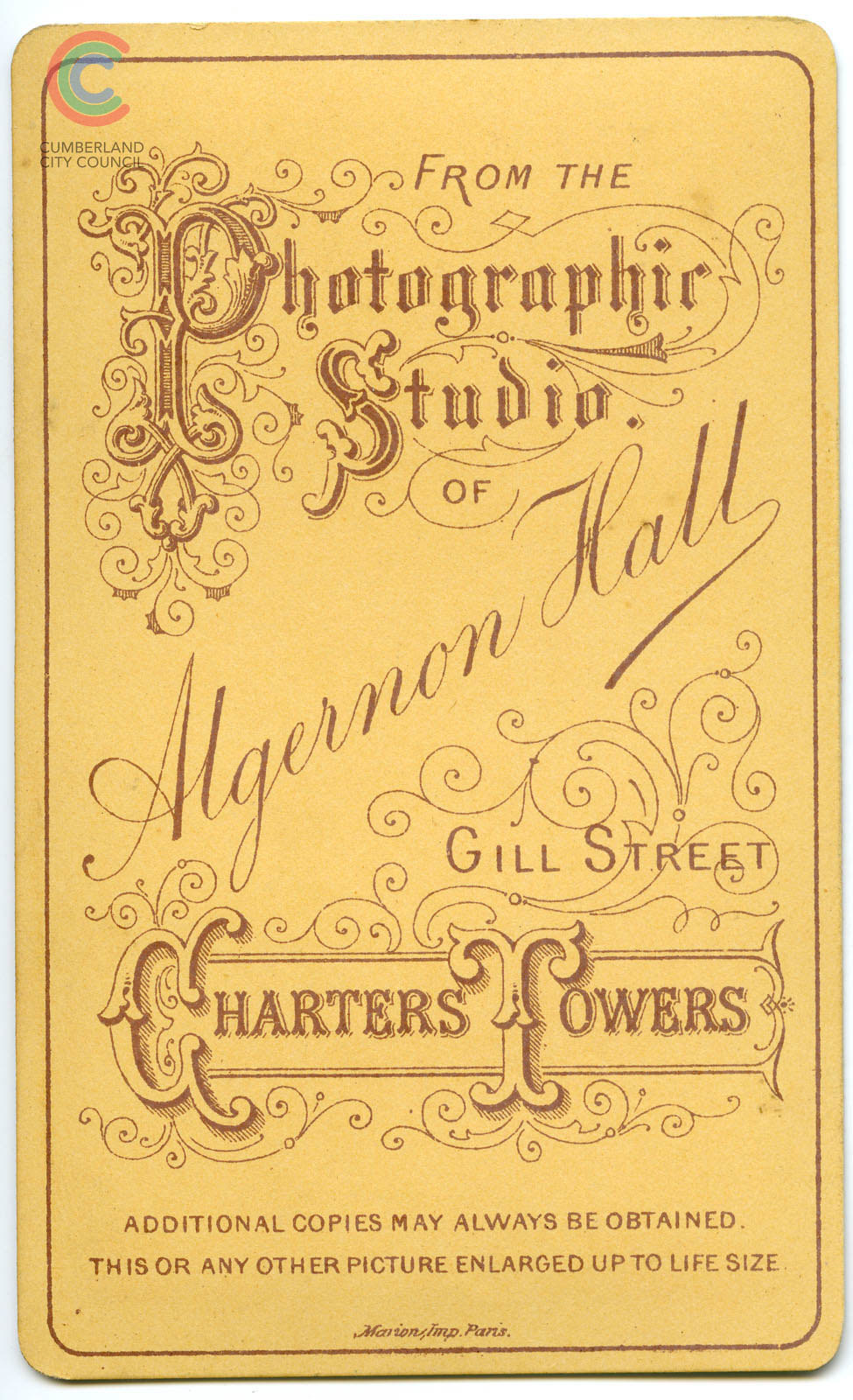The image depicts an aged, yellowed card that appears to be from the photography studio of Algernon Hall. The card, featuring a transparent white background, is adorned with an ornate, brown font that has faded over time. The heading "Photographic Studio" is written in highly stylized and decorative letters, while "Algernon Hall" is inscribed below in a more fluid, handwriting-like script that ascends at an angle. Further down, the card specifies the studio's location at "Gill Street, Charter Towers," and reassures that additional copies of photographs can always be obtained, with options to enlarge any picture up to life-size. At the bottom, the card notes "Marison's Imp. Paris," indicating the place of printing or import. The upper left corner of the image displays a logo featuring a blue C inside a green C inside a red C, labeled "Cumberland City Council." This logo appears to have been superimposed onto the card.